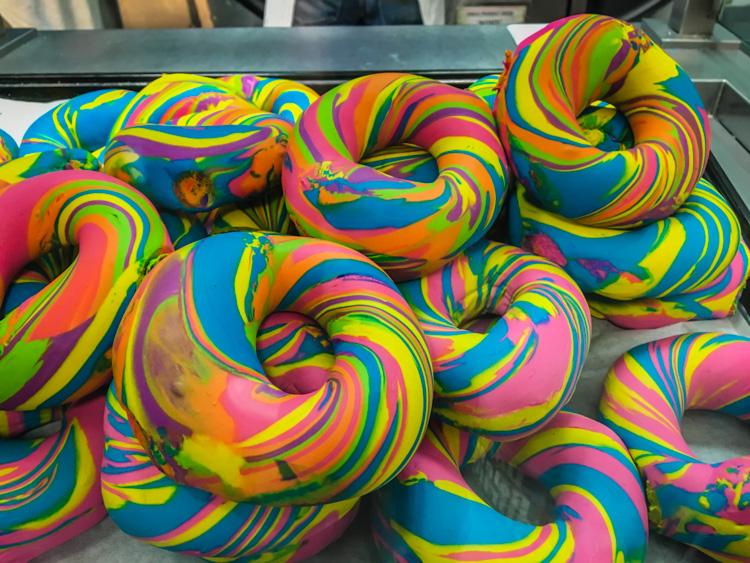The image showcases a vibrant, staged indoor scene under artificial lighting, which captures a collection of colorful, clay-like donuts stacked in tiers. These playful donuts, made from a squishy, Play-Doh-like material, feature swirling tie-dye patterns in shades of pink, yellow, blue, orange, green, and black. Each donut boasts a unique mix of colors and patterns, making no two alike. The setting includes a gray table and a similar-colored countertop behind the donuts. Partially visible in the background is a person wearing blue jeans and what appears to be a white lab coat, with the frame only capturing a section of their groin area. Additional background elements include what resembles a steel or aluminum bin and various boxes, adding to the scene's intriguing, staged composition.